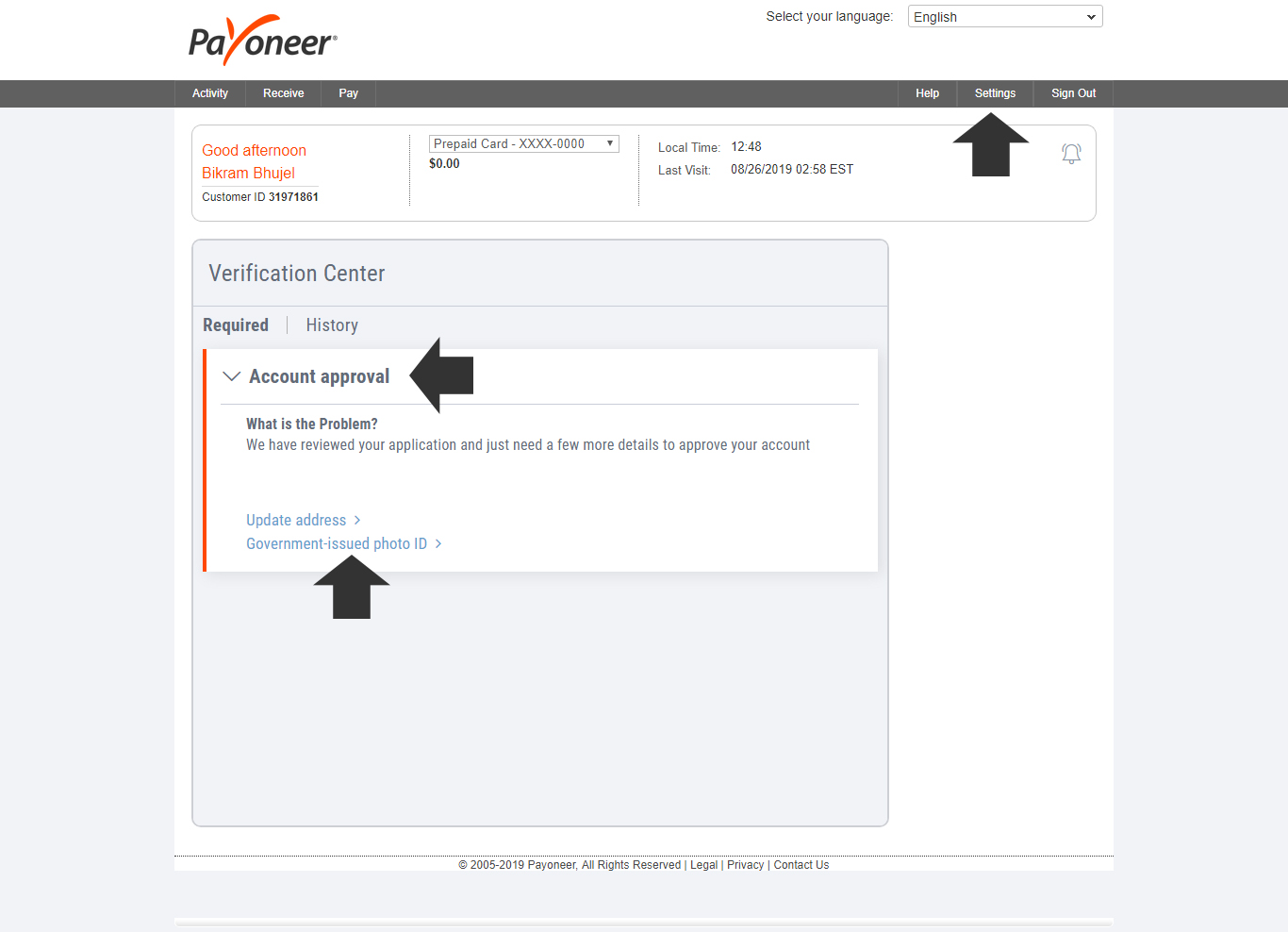This image is a screenshot from the Payoneer cash payment website. At the top of the page, there is a "Select Your Language" drop-down menu with English selected. Below this menu, a black navigation bar is visible, featuring tabs labeled "Activity," "Receive," and "Pay," as well as "Help" and "Settings" to the right, with an upward-pointing arrow highlighting the "Settings" option followed by a "Sign Out" link.

On the left side under the navigation bar, a greeting reads "Good Afternoon, Bikram Boydrell," along with the customer ID: 319-7861. To the right of this greeting is an outlined box displaying a prepaid card number partially obscured for security (XXXXXXX-0000) with an icon indicating there are no funds in the account. 

The current local time, 12:48, and the last visit, noted as August 26, 2019, at 02:58 EST, are indicated above a notification bell symbol on the right-hand side.

Below this section is the "Verification Center," which includes two tabs: "Required" (the currently active tab) and "History." In the active "Required" section, an account prompt titled "Account Approval" is present, highlighted by a left-facing arrow. The prompt includes a message stating: "We have reviewed your application and just need a few more details to approve your account." At the bottom of the section, there are options to update the address and submit a government-issued photo ID.